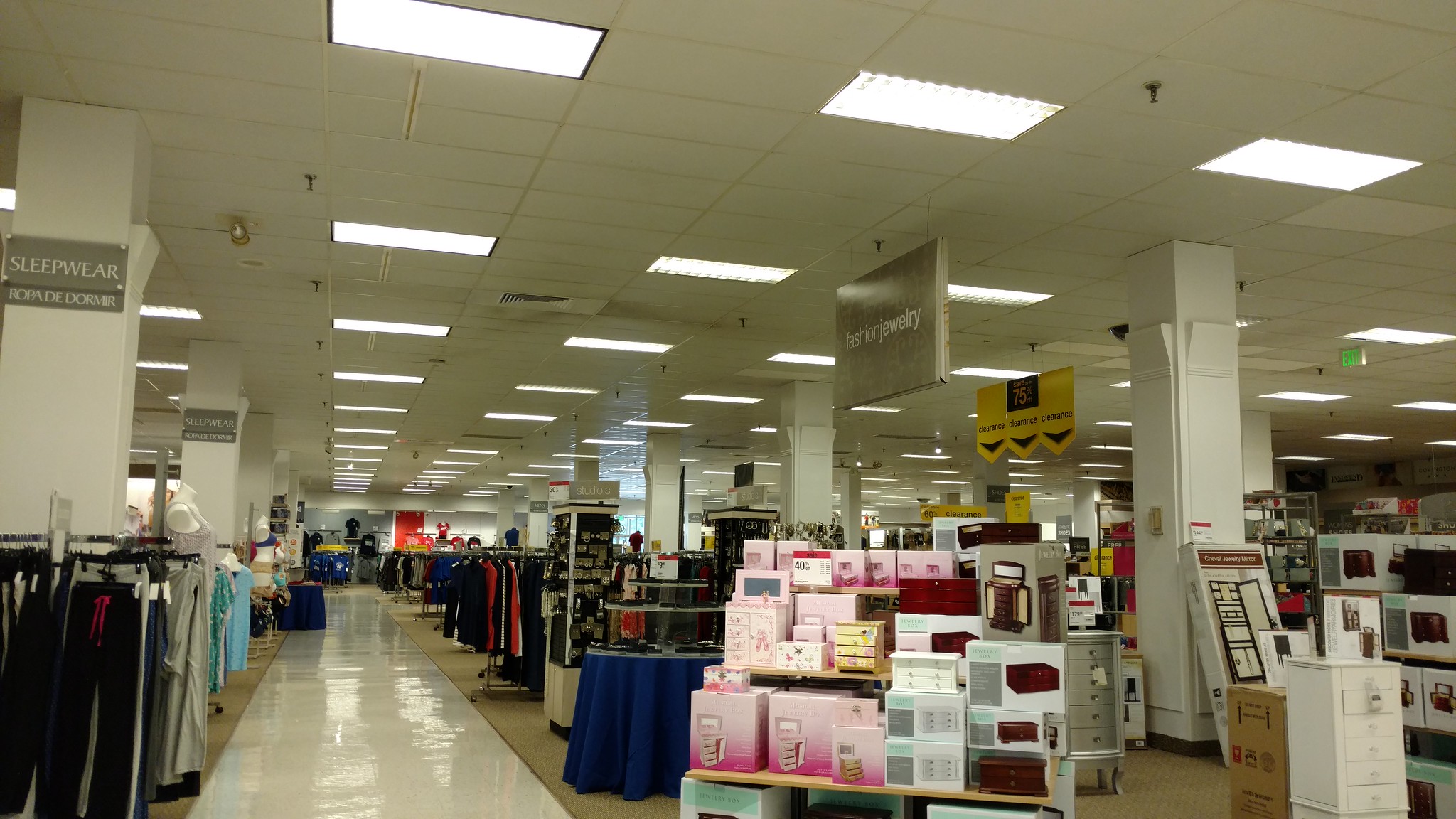In this rectangular, horizontally longer image of a department store, a shopper's viewpoint reveals a bustling retail environment with several sections and detailed displays. A long aisle, composed of shiny white tile, stretches from the near left side to the background, providing a pathway between two areas of merchandise. Overhead, white ceiling tiles are fitted with long, bright lights, illuminating the store beneath big yellow clearance signs pointing downward, boasting savings of up to 75%.

On the right side of the aisle, there's an array of household appliances and various items stacked in purple and gray boxes, alongside multiple stands displaying jewelry boxes in an assortment of colors. A prominent white stand with six small, clear-handled drawers sits further right, offering more jewelry storage options. A little round table covered with a blue tablecloth supports additional display items.

The left side showcases clothing, starting with racks of pants and moving toward a section featuring sleepwear, as indicated by a sign. A rounder holds sweatpants, while a mannequin dressed in a beige tank top hints at an adjacent lingerie department with another mannequin modeling a blue bra and tan underwear. Towards the end of the aisle, a gray wall displays men's polo shirts and t-shirts in the far back. The store is densely packed with varied stacks and racks of clothing, ensuring a wide selection for shoppers.